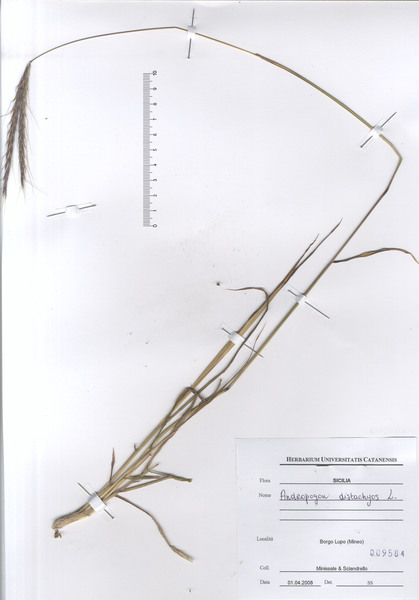The image depicts a dried plant specimen, likely some type of grass or wheat, meticulously arranged on a white sheet of paper. The plant, which appears to be in a premature state with small twigs branching out, is bent in the shape of the number 7 and features a distinctive curved tip with a bristle or brush-like end. It is securely taped and pinned to the paper, with a small, out-of-focus piece of text at the bottom right that likely contains the specimen's name and other scientific details. A ruler is also included on the paper, marked from 0 to 10 centimeters or inches, providing a scale to measure the plant, which is approximately 8 to 10 times longer than the ruler's scale. The specimen is carefully preserved, possibly for analysis or inclusion in a botanical database.